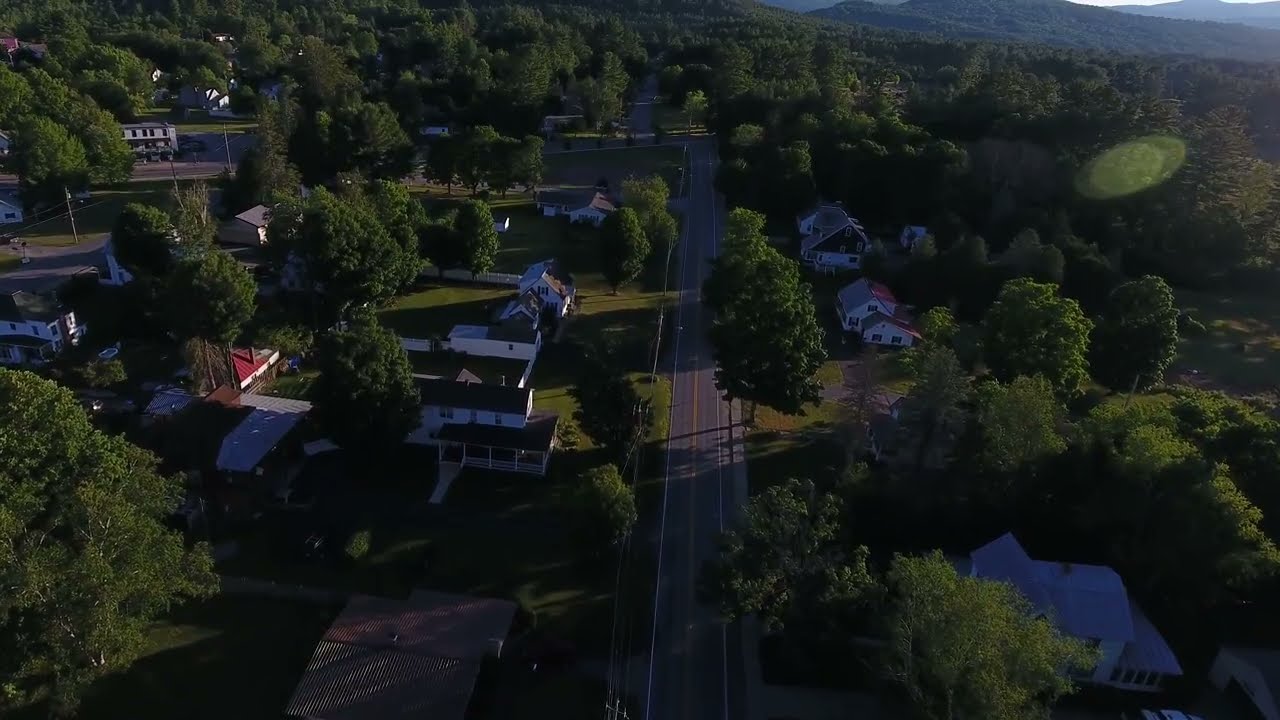This aerial view photograph, likely captured by a drone, showcases a picturesque small town nestled among lush, abundant greenery. The main focus of the image is a two-lane residential road running vertically through the center, flanked by a variety of homes ranging from ranch-style to two or three-story houses. The houses, varying in architectural design and made largely of wood, are surrounded by dense trees and foliage, contributing to the overall verdant appearance of the community. 

On the left and right sides of the road, numerous substantial homes—some potentially as large as 4,000 to 5,000 square feet—can be seen with driveways, although no cars are visible on the road itself. In the lower right section of the photo, there might be a body of water or perhaps a reflective surface, adding a unique element to the landscape. 

In the distance, the image reveals a serene background of rolling hills and mountain ranges, with a glimpse of clear, sunny sky above, indicating perfect weather conditions. This blend of residential charm and natural beauty encapsulates the tranquil essence of this tree-covered, suburban community.